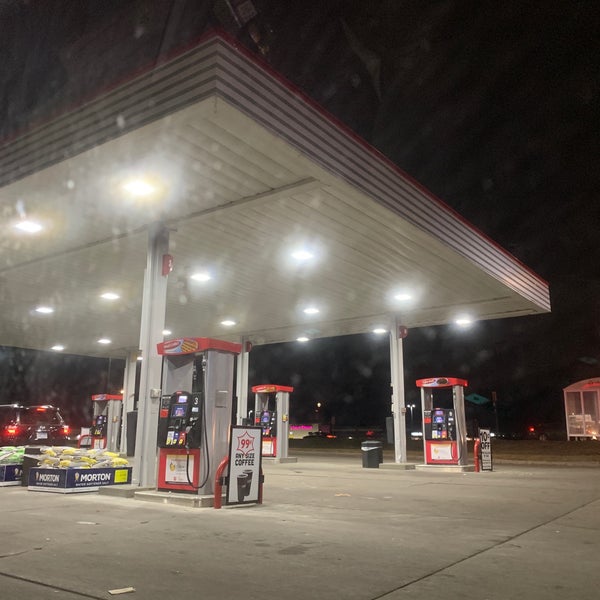This nighttime photograph captures a gas station scene viewed through a dirt-streaked glass surface, which reflects some ambient lights. The main focus lies on the brightly lit gas pumps framed by a red, gray, and white overhang. The pumps are designed in matching red, white, and black colors. Beside one of the pumps stands a sandwich board advertising "99¢ coffee" in bold red and black letters, illustrated with images of steaming coffee cups. An additional signboard with black font displaying various numbers and letters is also visible. Black trash cans are strategically placed around the area, contributing to a somewhat cluttered environment. A dark-colored vehicle with illuminated red taillights can be seen in the background. The scene includes a stack of Morton ice melt bags positioned near the concrete ground, adding to the utilitarian atmosphere of the gas station at night.